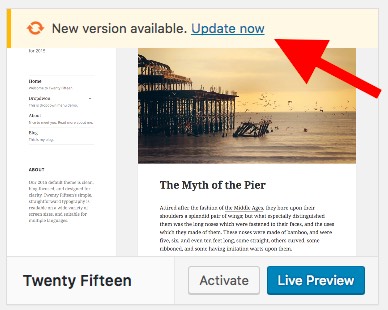This desktop screenshot features a predominantly gray background with narrow light gray margins. At the center of the image is an orange refresh button accompanied by the text "New Version Available" and a blue hyperlink that says "Update Now." A red arrow, originating from the bottom right-hand corner and directing to the left, points diagonally to the "Update Now" link. The surrounding background of this section is a light flesh tone.

Below this notification, there is a captivating image of a pier extending into a vast ocean, with a flock of birds soaring in the background. In the middle of the water, a jet ski can be seen skimming the surface. The pier, an open-air structure, is supported by numerous pillars.

Below the image, the phrase "The Myth of the Pier" appears against a white background. Although the accompanying text is unreadable, the date "2015" is clearly marked on the extreme left at the bottom. To the right of the date, two buttons are visible. The first button, colored white, is labeled "Activate," while the second, in navy blue, reads "Live Preview."